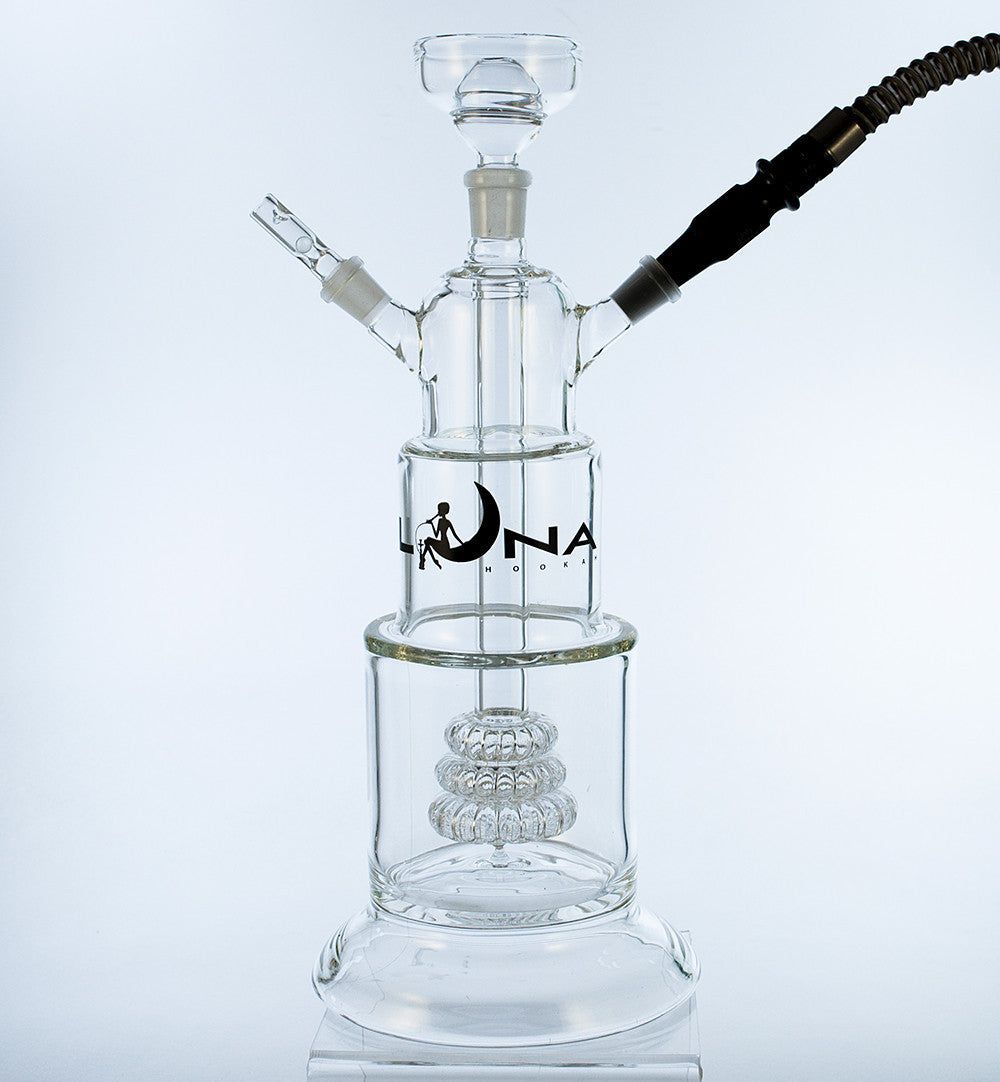The image showcases an elegant, high-tech hookah by Luna Hookah. This sophisticated device is crafted from transparent glass and follows a multi-tiered structure with three stacked cylinders. The base is large and round, transitioning into a flat surface before ascending into another cylinder, and finally another flat surface leading to the top cylinder. The hookah features a Luna Hookah logo in black, with a distinct "U" represented by a crescent moon with a person sitting on its edge. Notably, the hookah is fitted with a glass bowl at the top for the shisha and includes a black hose for smoking. Intricate details like a pyramid formation of bead-like structures inside one of the cylinders add to its modern and expensive appearance. The hookah is accompanied by black tubing extending from the right and left sides, contributing to its elegant and refined look.